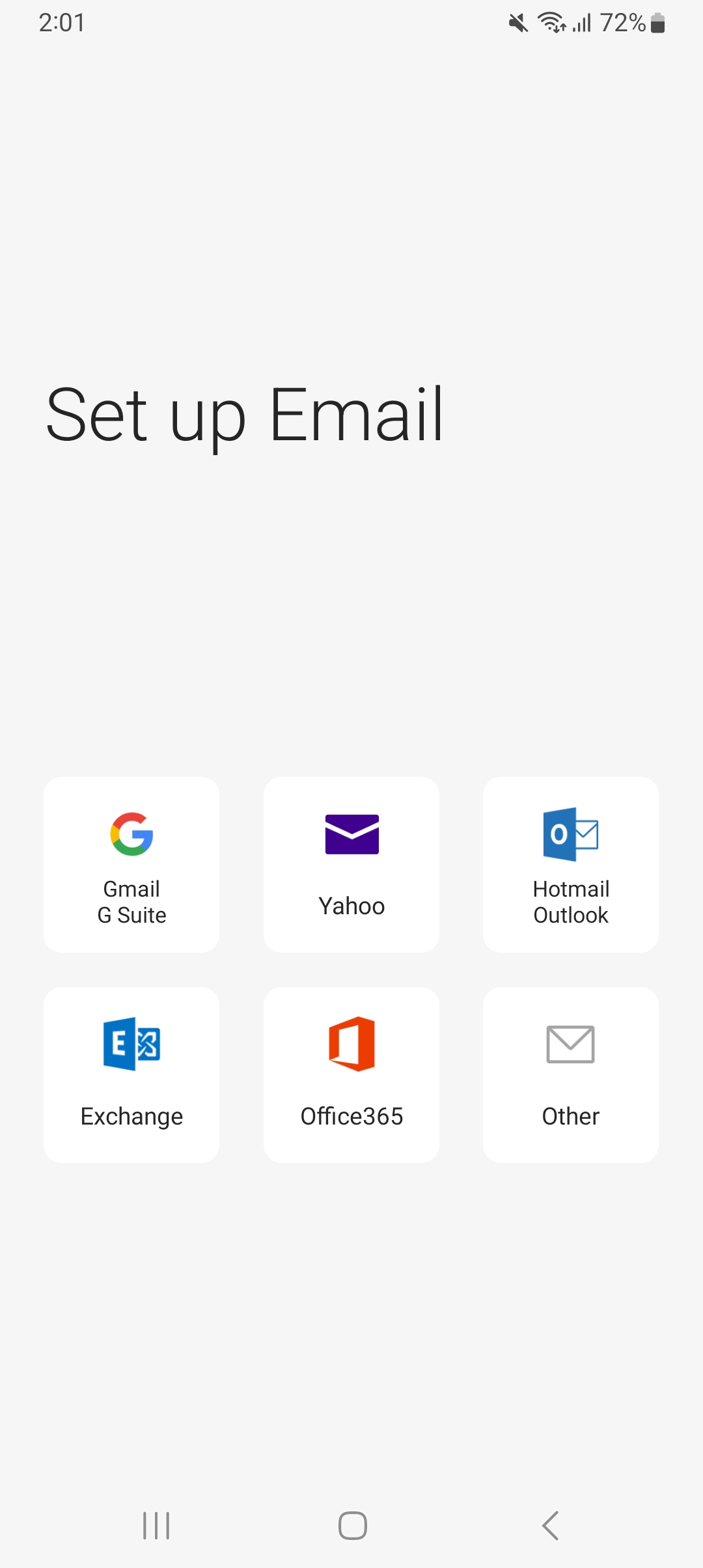Screenshot showing a smartphone screen with detailed information. The phone displays the time as 2:01 and shows full signal strength with a 72% battery level. The background is an off-white shade. At the top, prominent text reads "Set up email." Below this heading, there are six white boxes laid out against the off-white background, each representing an email service option:

1. **Gmail/G Suite:** Marked with Google's emblem.
2. **Yahoo:** Displayed with a blue envelope icon.
3. **Hotmail:** Featuring a half-envelope combined with a half-teal square with a white circle inside.
4. **Exchange:** Identified by an 'E' and a barcode symbol.
5. **Office 365:** Represented by a red square with an open center.
6. **Other:** Depicted with a generic envelope icon.

Each email service is distinctly presented with its respective logo or symbol for easy identification.